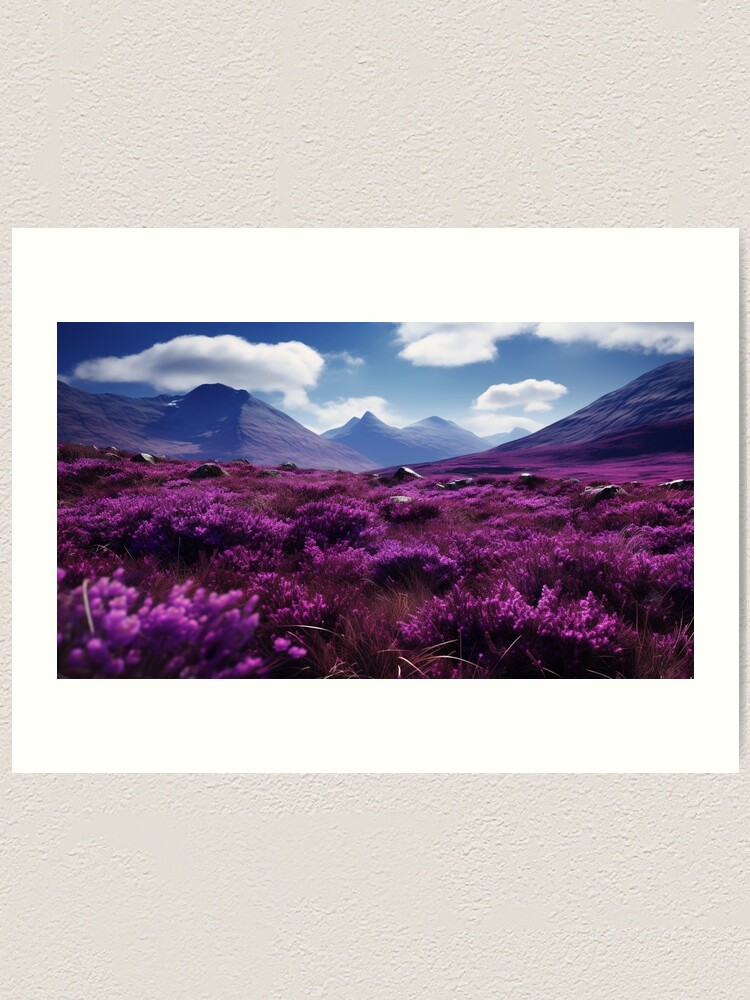The photograph, mounted on an off-white, lightly textured wall, is a professional piece of wall art set in a landscape-oriented white frame with a thicker top border. It captures a breathtaking outdoor scene featuring a vibrant blue sky dotted with floating, cotton-like white clouds hovering above a series of bluish-purple mountains. The foreground is dominated by a sprawling field of vivid lavender flowers, their rich hues stretching from the middle of the image to the bottom, creating a seamless and striking contrast against the sky and mountains. The overall composition, framed with a white border, is visually striking, showcasing deep, vibrant shades of purple, magenta, and blue, with grayish tones accenting the mountains, making it a captivating and serene depiction of nature.